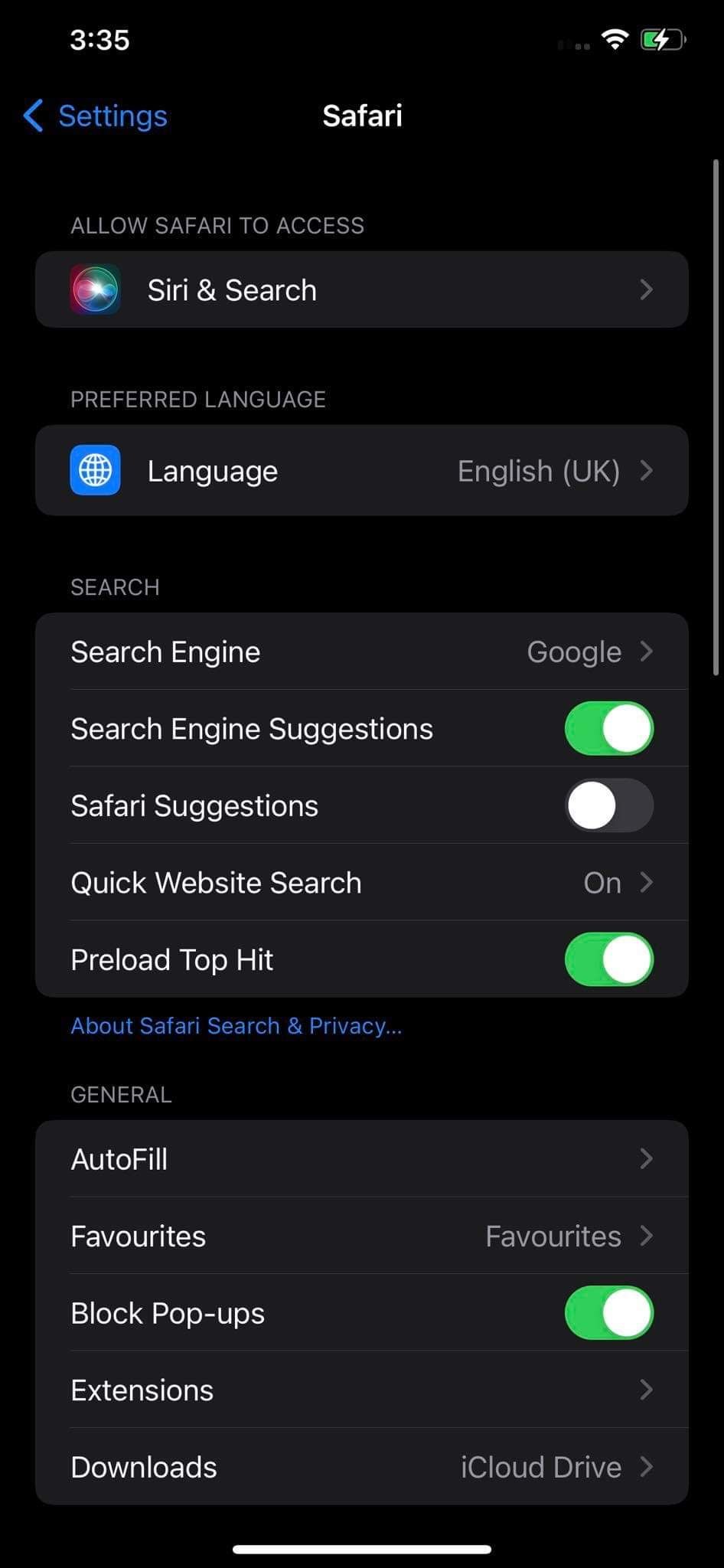The image is a screenshot taken from a mobile device's settings menu, predominantly featuring a black background. The screenshot was captured at 3:35, as indicated by the time displayed at the top of the screen. The carrier signal shows no bars, but the device is connected to Wi-Fi. The battery icon indicates the device is charging and is currently at approximately 50% capacity.

At the top of the screenshot, the word "Settings" appears in blue, accompanied by a left arrow for navigation. The central focus of the screen is the settings for the Safari browser. The header "Allow Safari to Access" is visible, followed by various customization options.

The first option, "Siri & Search," is available for selection. The preferred language is set to "English (UK)." The search engine is set to Google, and the toggle for "Search Engine Suggestions" is switched on, indicated by a green switch. In contrast, the toggle for "Safari Suggestions" is turned off.

Other settings visible include "Quick Website Search," which is enabled (green toggle); "Preload Top Hit," also enabled with a green toggle; and "Autofill," "Favorites," and "Block Pop-ups," all of which are turned on, as indicated by their green toggles. Additionally, there are options for "Extensions" and "Downloads" visible towards the bottom of the screen.